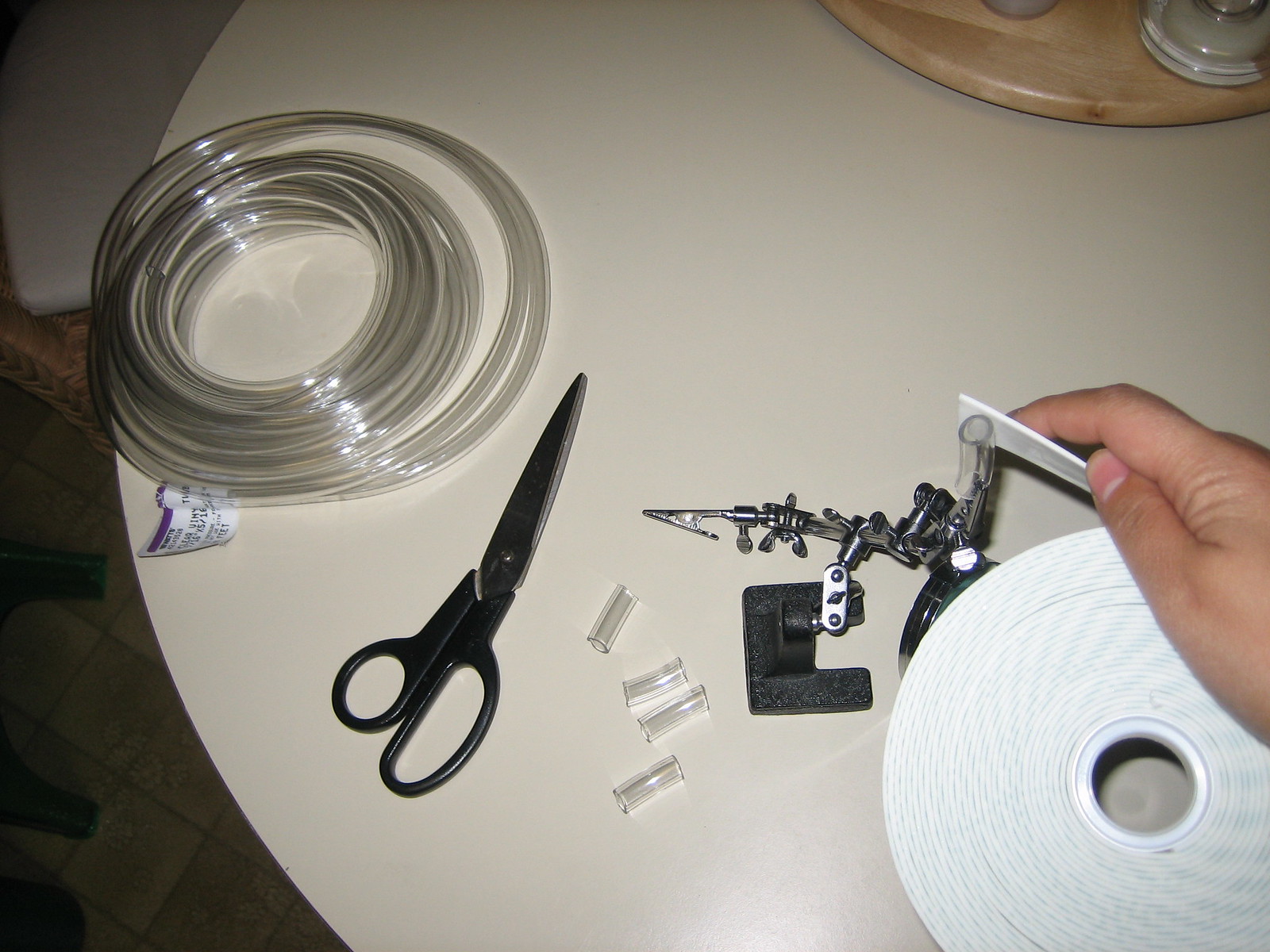The image depicts a white table on which a person is engaged in a small project involving the cutting and wrapping of clear hose, seemingly fish tank hose. The upper left corner of the picture shows a long coil of this transparent hose neatly curled. Nearby, a pair of heavy scissors with black handles lies adjacent to four small cut pieces of the same hose. To the right of these cut pieces, a stand and clamp apparatus is set up, securing a length of hose. The person's hand is visible in the frame, holding what looks like a roll of insulating tape, indicating their intention to wrap this tape around the section of hose held in the clamp. The scene captures the meticulous nature of the task and the array of tools and materials involved in this detailed DIY project.